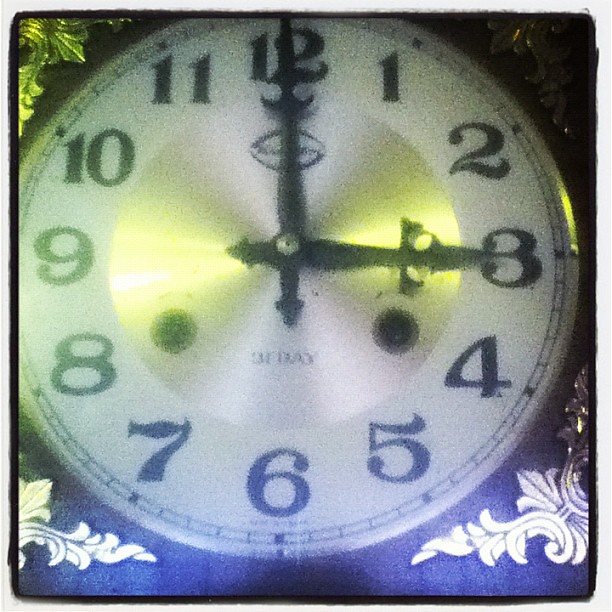This is a detailed close-up photograph of a vintage, ornate clock housed in a square case with a black background and elaborate metallic floral and leaf designs in each corner. The clock's white round face is contrasted by bold, black numerals in an ornate style, circled by a silver inner ring. The minute hand points at 12 while the hour hand is at 3, indicating 3 o'clock. Positioned within this silver ring are two small black holes for winding the clock, requiring special keys. Small notches between the numbers allow for precise time reading. There is a partially obscured brand signature near the bottom, and a symbol near the 12 that is hidden by the minute hand. The entire clock assembly is mounted on a piece of rich, dark chocolate brown wood with intricate metallic trellising in each corner, enhancing its classic, elegant appearance.